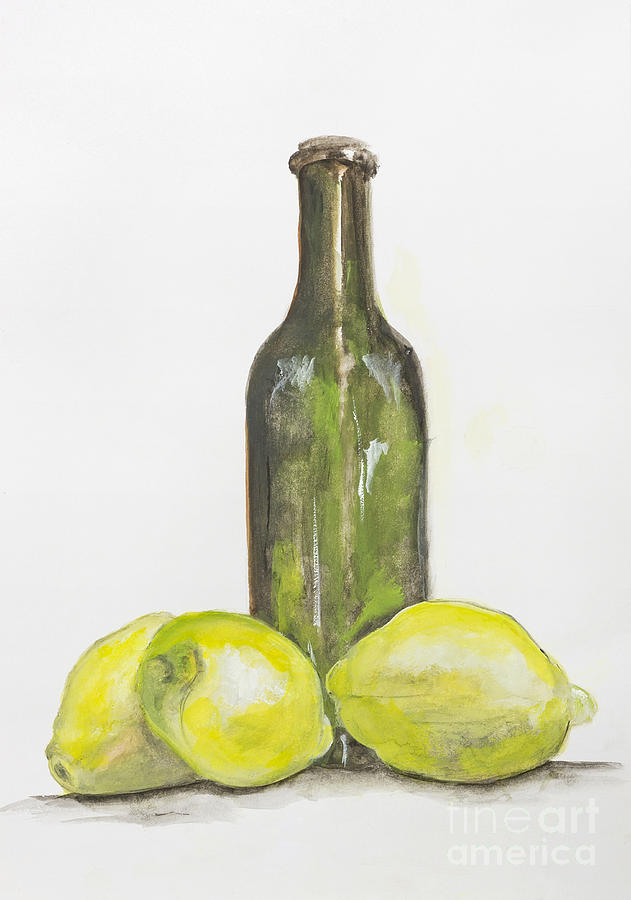This image is a detailed watercolor or acrylic painting titled "Fine Art America," faintly inscribed in white letters in the bottom left corner. The painting depicts a tall, antique-style glass bottle without a stopper, situated centrally. The bottle, in shades of green—ranging from brownish-green to lime green—features reflections and light smudges that may represent small flowers. In front of the bottle are three sizable lemons, varying from bright yellow to paler shades, with white highlights and green at the tips. The background is predominantly off-white, creating a stark contrast to the pale tannish surface on which the bottle and lemons rest. The overall style is illustrative with a focus on light and shadow, capturing the reflections on the bottle and the subtle textures on the lemons.